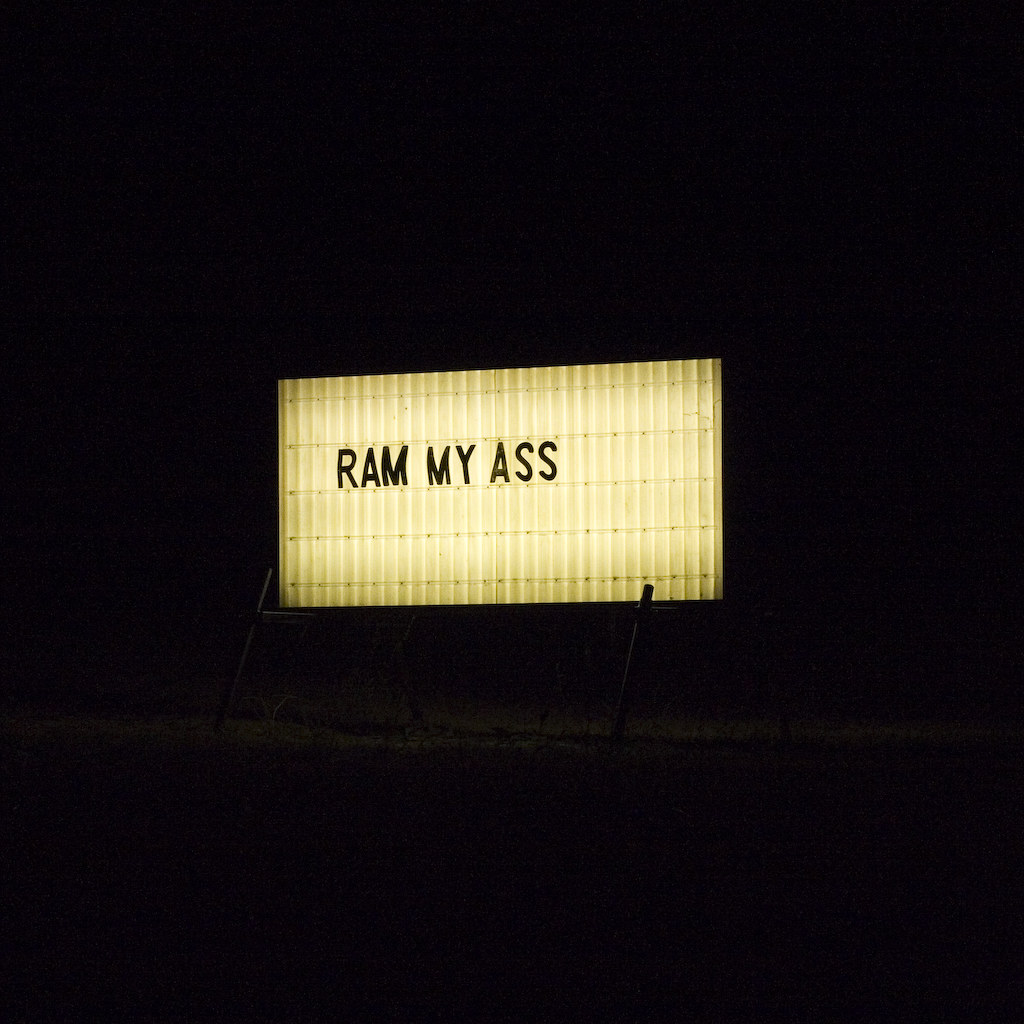The image depicts a rectangular, yellow marquee billboard outside at night, standing out starkly against a pitch-black background. This sign, illuminated by dim backlighting, reveals its structure, showcasing vertical grooves and horizontal bars, faintly visible due to the light. The text on the sign, composed of black capital letters arranged by hand, spells out the phrase "RAM MY ASS" in the center. Clearly intended as a prank, the message stands in sharp contrast to the surrounding darkness, making the otherwise hidden frame of the sign slightly perceptible.